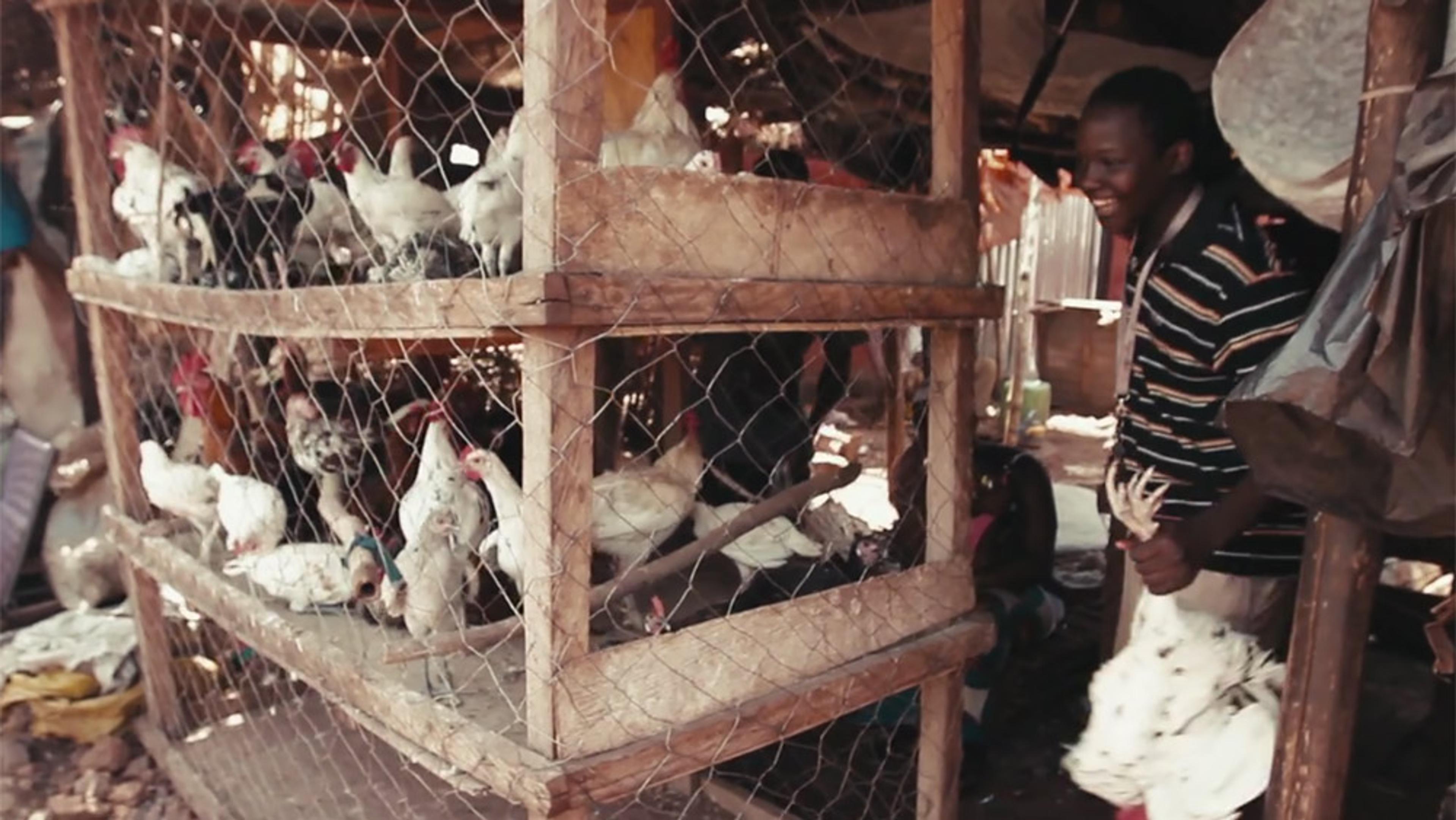In this outdoor scene, a smiling African man stands beside a three-tiered wooden chicken coop encased in thin metal chicken wire. The coops, possibly homemade, are filled with smaller-sized chickens, predominantly white and speckled, along with a rooster or two. Each level of the coop, measuring roughly five feet in length and three feet in width, houses around eight chickens. The bottom level appears empty, while the top two levels are occupied. The man, dressed in a black and red striped shirt, is laughing heartily as he holds a chicken upside down by its legs in his left hand. The sunny setting suggests a rural village, potentially in Sub-Saharan Africa, where chickens are kept for food. The photo, taken with its head cut off, leaves the life status of the chicken in the man's hand unclear.